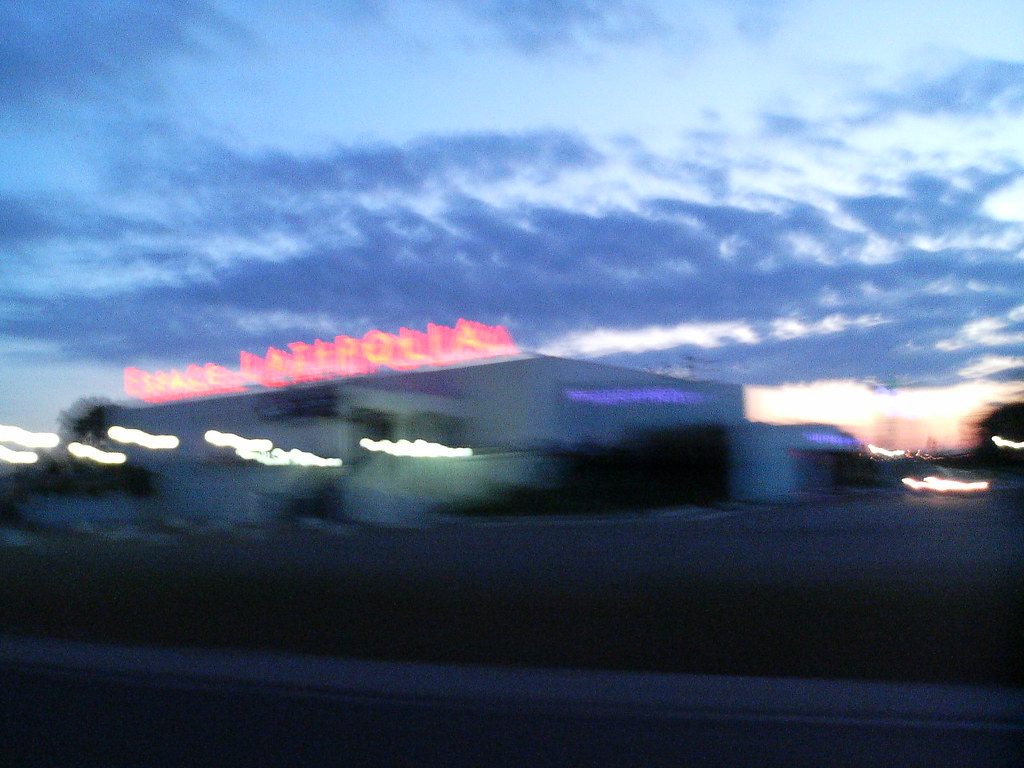This image is a rectangular, nighttime outdoor photograph of a slightly blurry establishment, likely a store. The building runs horizontally across the image, starting near the left center and extending about three-quarters of the way to the right. The structure is oriented towards the left, revealing its right corner and part of its front facade.

The building appears to be one or two stories tall, constructed from a white stone or brick material. At the top, there is a brightly lit, orange-red sign displaying a five-letter word that is challenging to read, possibly "ESSACE," followed by "LATIRLOLIA," which may be in a different language.

Lavender lights are visible near the right side of the building, with one light positioned across the entryway and another slightly further back on the wall. In front of the building lies some shrubbery, and the scene opens up to a mostly empty parking lot characterized by a large gray area, suggesting the location may be part of a shopping mall or plaza.

To the right side of the building, there are some red and white lights, likely from parked automobiles. The sky features dark blue clouds, indicating the sun is setting, with some bright white areas peeking near the horizon in the back right, contributing to the twilight ambiance.